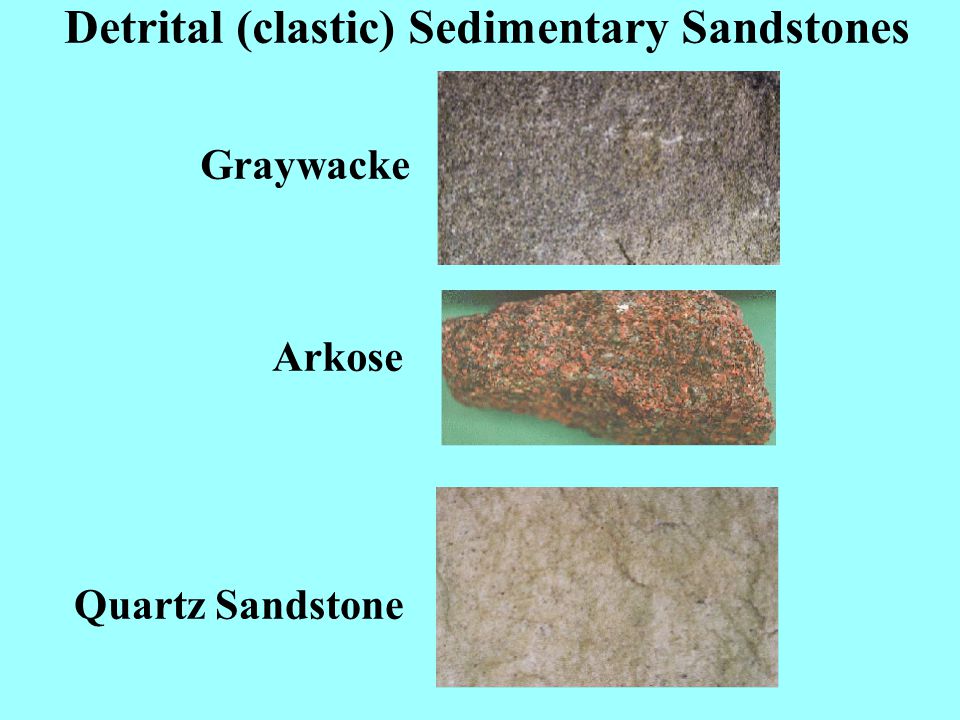Against a light blue background, the image features the bold black text "detrital (clastic) sedimentary sandstones" at the very top. Down the left side, labels identify three types of sandstone with accompanying photographs to the right of each label. 

At the top, "Greywacke" is labeled beside a grey stone speckled with white. Below this, "Arkose" is labelled next to a rock characterized by orange, brown, and white hues; the stone rests on a green surface. At the bottom, "Quartz Sandstone" is labeled next to a close-up image revealing a predominantly white sandstone interspersed with grey and dark green veins. Each rock is enclosed within a rectangular frame. The detailed, academic presentation suggests this image is designed for educational purposes.